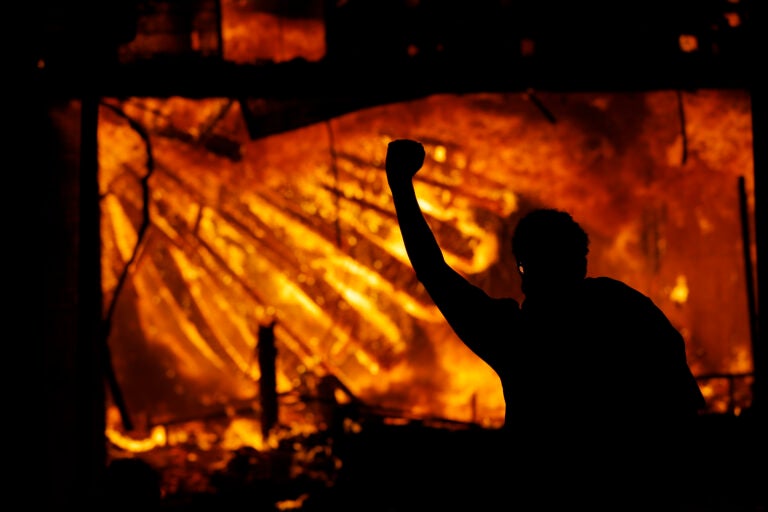The photograph captures a striking silhouette of a person standing with one fist raised triumphantly above their head, located in the right half of the image. This person appears to have short, fluffy hair and an uneven shape, suggesting they are either draped in a cape or carrying a bag over their back. Their silhouette is the only element in focus against an out-of-focus backdrop of glowing orange and yellow hues, which are interspersed with diagonal slanted lines and a black border. This backdrop gives the impression of a burning building, accented with debris and structural elements like collapsed sections and wires. The intense, fiery colors—primarily black, red, orange, and yellow—create a vivid and dramatic scene, often associated with night-time. The overall atmosphere evokes a sense of triumph or exclamation amidst chaos, as the person stands in sharp contrast against the blazing background.